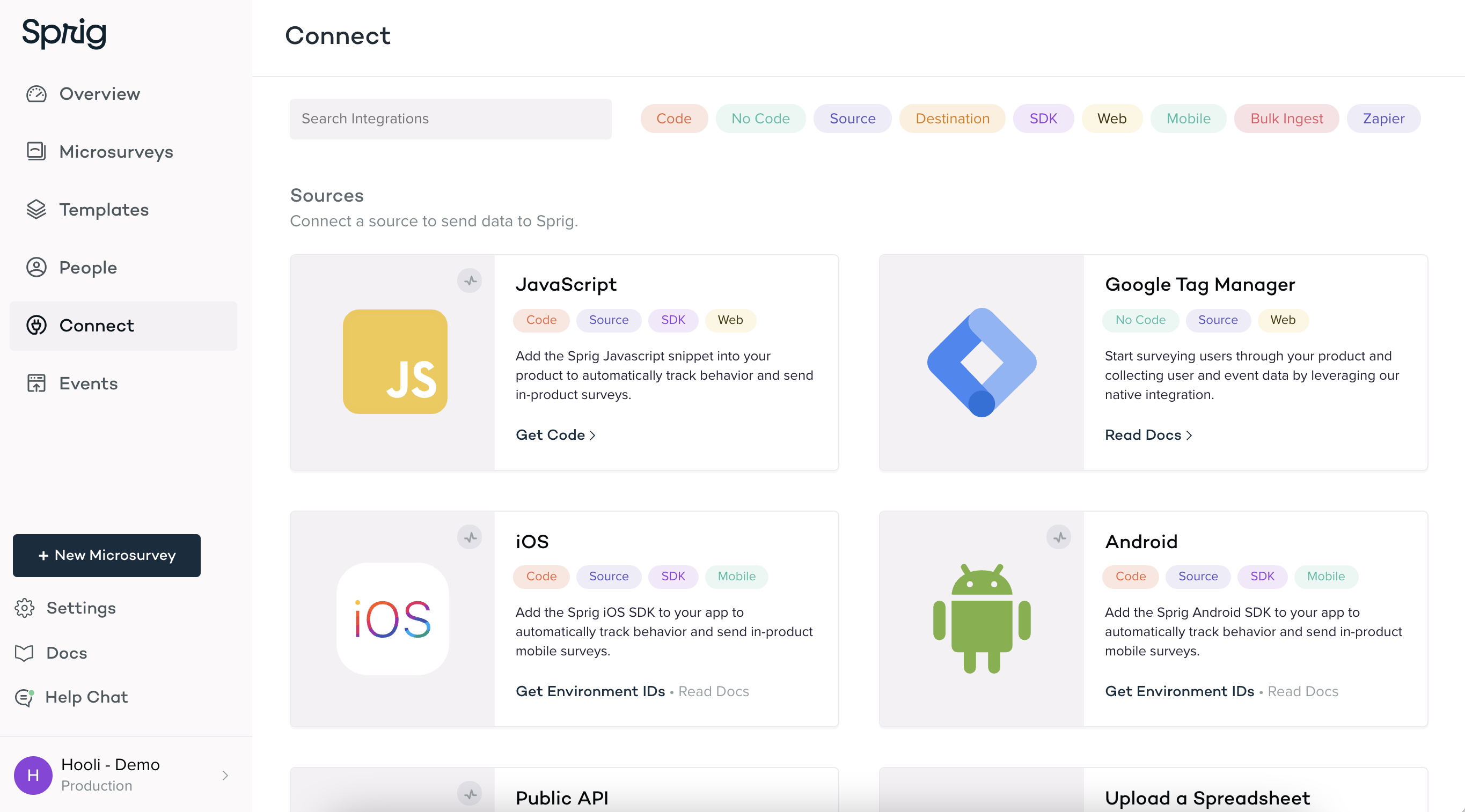Screenshot of Sprig's interface showcasing a variety of menu options and functionalities. At the top, tabs include 'Overview,' 'Microsurveys,' 'Templates,' 'People,' 'Connect,' 'Events,' 'New,' 'Microsurvey,' all with a highlighted blue rectangle behind 'Microsurvey.' On the right, there are additional options such as 'Settings,' 'Docs,' 'Help Chat,' and a search bar labeled 'Search Integrations.' Below, integrations are categorized under 'Code,' 'No-Code,' 'Source,' 'Destination,' 'SDK,' with options for 'Web,' 'Mobile,' 'Bulk Ingest,' and 'Zapier.' A section titled 'Sources' instructs users to 'Connect a Source to Send Data to Sprig,' listing integrations like 'JavaScript' (labeled with 'Code,' 'Source,' 'SDK,' and 'Web'), 'Google Tag Manager' (labeled with 'No-Code,' 'Source,' and 'Web'), 'iOS' (labeled with 'Code,' 'Source,' 'SDK,' and 'Mobile'), and 'Android' (similarly labeled with 'Code,' 'Source,' 'SDK,' and 'Mobile'). Two additional, partially visible options include 'Public API' and 'Upload a Spreadsheet.'